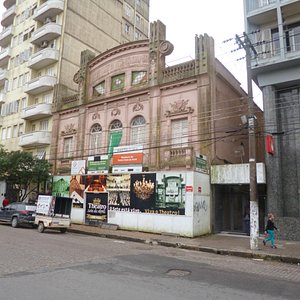The image depicts a detailed street view in an urban area featuring an older, ornate building constructed from reddish stone, with notable architectural elements possibly in the Art Deco style. The building, several stories tall, features intricate facade details including arched windows in the middle section, stone railings, and a high central panel that is curved. The building's lower portion is adorned with multiple posters, and a plywood structure, possibly for remodeling purposes, is present out front. Additionally, several decorative towers and relief stonework embellish the structure. 

In the foreground, there is a street with a curb, where a small van is parked, sporting a two-wheeled trailer. To the left of the main building is a taller, yellowish stone apartment building with balconies, and to its right is a portion of another, bluish stone building cut off from the frame. A prominent light pole with atypical electrical connections stands close to the main building. The image captures not only the architectural grandeur of the primary building but also the diverse urban environment, providing a glimpse of typical city life with vehicles and mixed architectural styles.